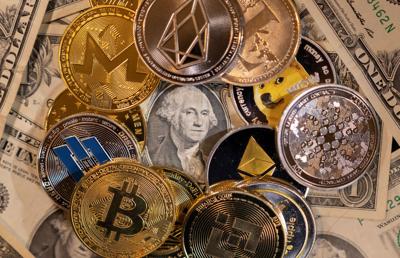The image showcases a meticulously arranged composition of currency, featuring a backdrop of overlapping one-dollar bills with a prominent close-up of George Washington's face as the centerpiece. Surrounding this central figure is a ring of various cryptocurrency coins. Among the eight to ten coins, one prominently displays the Bitcoin symbol with a 'B' and vertical lines. Other coins include those with symbols like a large 'M', a stylized 'L', a geometrical diamond shape, a square shape, and a coin featuring the internet-famous Doge meme. These coins range in colors from gold to silver to bronze, including a distinctive black coin with a gold pyramid and another with a canine figure. The dollar bills are intricately crisscrossed, adding depth and texture to the background, all subtly reflecting the number one and the words "one dollar." This artwork elegantly juxtaposes traditional fiat currency with modern digital assets.